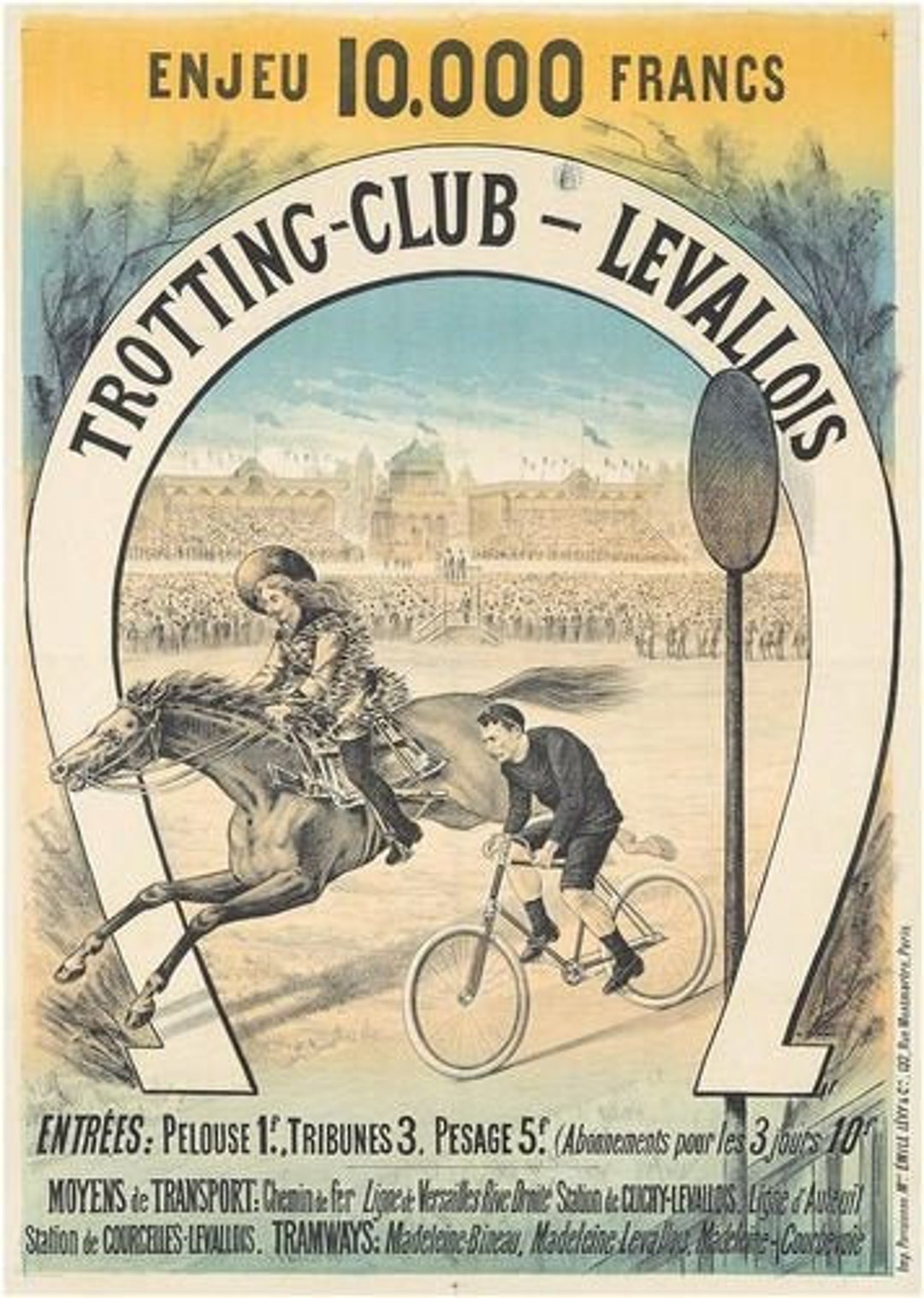The image is a rectangular, printed material in French, measuring approximately six inches in height and three to four inches in width. It features a thin, light tan border surrounding the main contents. At the top, in a section with a faint dark yellow background transitioning into light blue, the text "Enjeu 10,000 francs" is prominently centered in black print. The first word is spelled E-N-J-E-U.

Below this, the background depicts tree branches flanking the sides and transitions into a bustling scene. At the heart of the image is a large brown building resembling a castle, set behind an arena teeming with people. In the foreground, a detailed drawing shows a woman riding a horse on the left side, and a man riding a bicycle to her right, appearing as though they are in a race.

Surrounding these figures is a prominent white horseshoe shape, inside which is the text "Trotting Club Levallois" in black print. Towards the bottom, over a blue background, additional French text reads "Entrees Pelloux 1, Tribunes 3, Passage 5," followed by more fine French lettering providing further details.